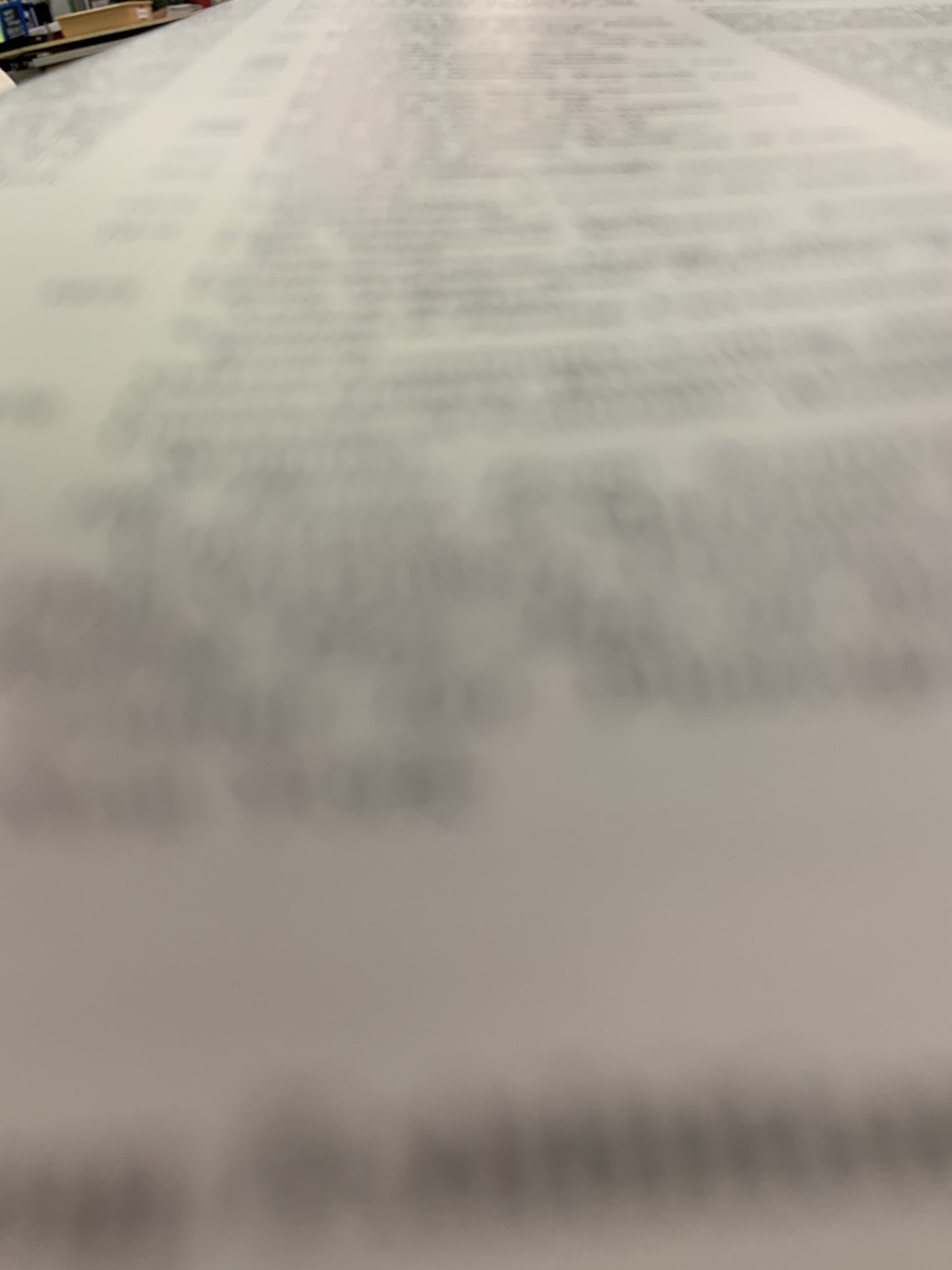This image presents an extremely close-up view of text, possibly from a page of a book or a script. The perspective is so zoomed in that the individual letters are blurred and illegible, rendering it impossible to decipher any specific words. The layout suggests a structured format; on the left margin, text is arranged as a column. A slight white space separates this column from more text, hinting at a narrative format typical of a story or script. Although the precise content remains obscured due to the blurring, the dense black markings indicate a significant amount of written material on the page.